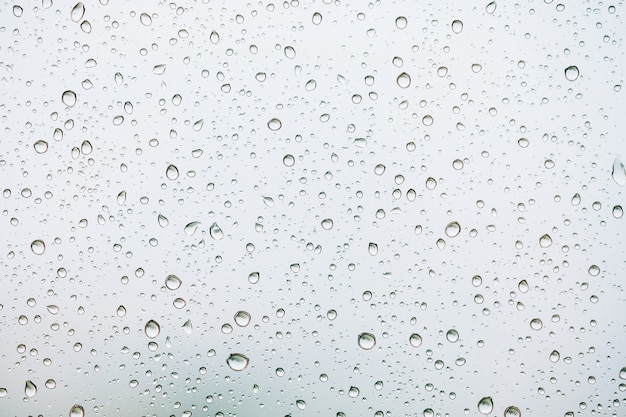The image displays a close-up of a window or sheet of glass covered in hundreds of water droplets against a gray, overcast backdrop. The water droplets vary in size and shape, ranging from tiny pinhead specks to full, larger raindrops, all of which are generally round and clear. Their texture and positioning suggest they are slowly dripping down the glass, giving an impression of motion frozen in time. The background is a soft gray that darkens slightly towards the bottom left of the frame, emphasizing the droplets' transparency. The overall scene evokes a quiet, gloomy atmosphere typical of a cloudy, rainy day, with no other colors present but shades of gray, white, and black.